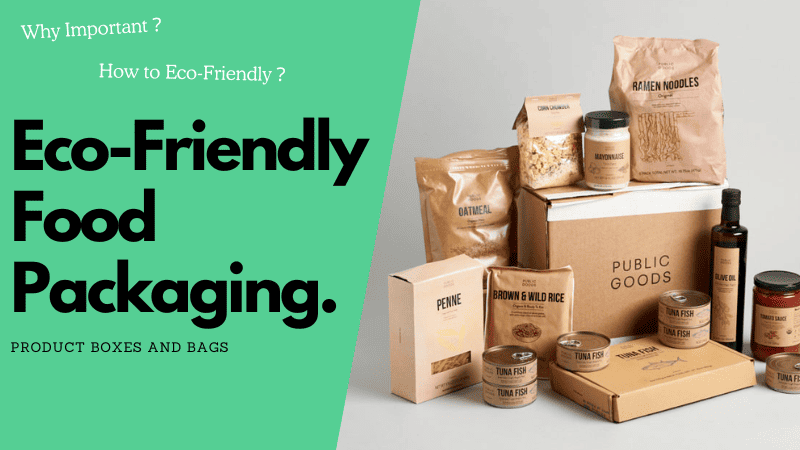The image is a rectangular advertisement, approximately six inches wide by three inches high, divided into two sections. On the left side, against a green background, white text poses questions: "Why Important?" and "How to Eco-Friendly?" Beneath these, in bold black font, it reads, "Eco-Friendly Food Packaging," followed by "Product Boxes and Bags" in smaller black print. On the right side, set against a light gray background, a variety of food products are shown, all packaged in eco-friendly materials. Central to this section is a large brown box labeled "Public Goods." Surrounding this box are various items, including a brown bag of ramen noodles, a jar labeled "Mayonnaise" with a black lid, a clear plastic bag with a brown top containing another type of noodle, a large bag of oatmeal, a small box of penne, and a bag of brown and wild rice. Additionally, there are six cans of tuna fish, a box of tuna fish, a jar of olive oil, and a jar of tomato paste. The assortment of packaging—boxes, cans, jars, and bags—highlights the commitment to eco-friendly food storage solutions.